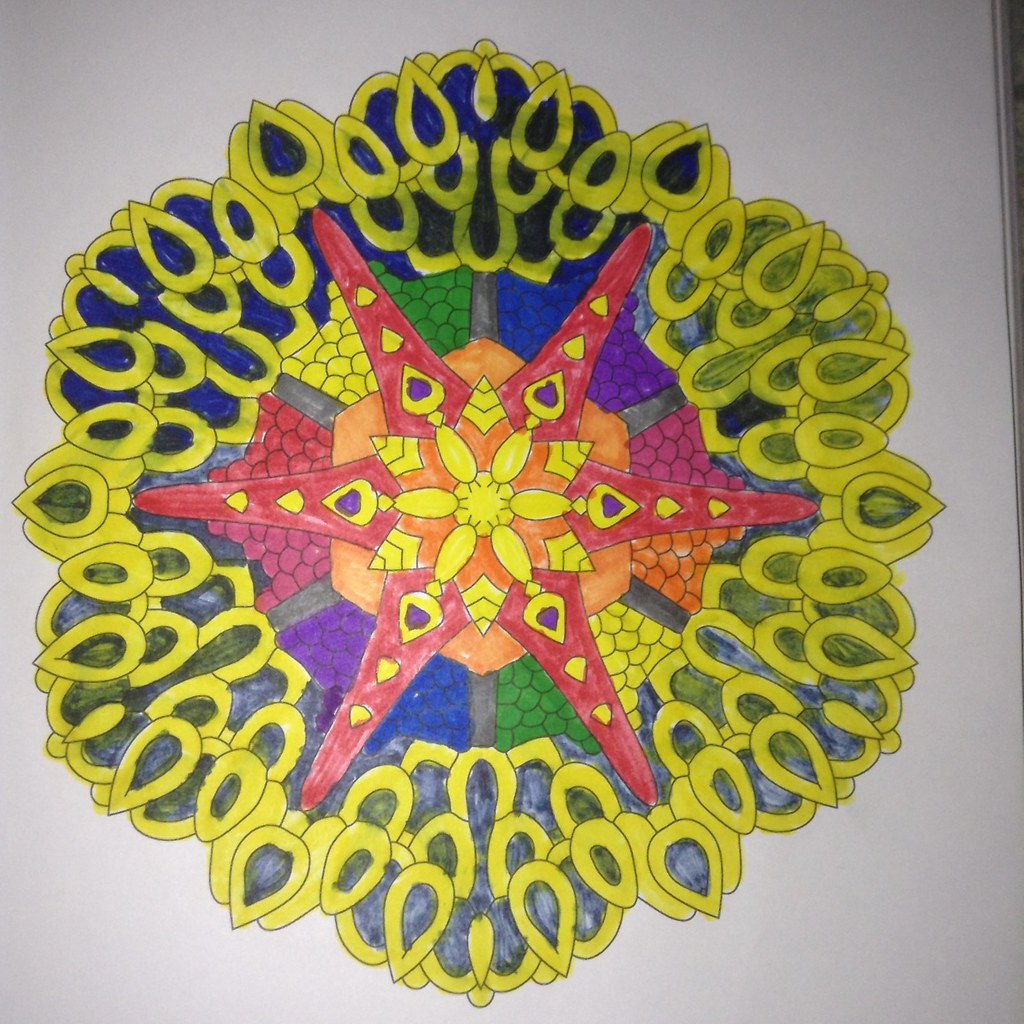The image is a hand-drawn and colored Mandela design on a white piece of paper, characterized by its intricate and multi-layered geometry. At the center of the design is a six-pointed star that combines yellow and orange hues with black lines forming V shapes. This central star is interlaced with another star shape, creating a complex inner structure where radial black outlines connect to yellow ovals and form a fragmented star pattern within a circle.

Surrounding the central stars, triangular pieces filled with purple hues and diamond shapes extend outward. Large red triangles, each topped by smaller yellow and purple triangles, create a 3D effect along the six points. These are spaced out evenly and contribute to the star's dynamic appearance. Below each triangle are sections with crown-like shapes in various colors, arranged in a sequence that includes pink, red, yellow, green, blue, and purple, adding to the richness of the design.

Encircling this central arrangement is a starfish-like pattern that integrates additional colors like pink, green, and blue, framed by teardrop shapes outlined in gold. These teardrop elements, with mixed interiors of dark blue, black, and gray, cascade outward further enhancing the complexity of the image. The outermost patterns radiate into leaf-shaped motifs that are predominantly yellow and blue, although the blue sections appear streaky due to fading ink.

The entire drawing is outlined with black ink and is vividly colored using felt pens, although some shading and coloration appear uneven due to ink inconsistencies. The careful layering of shapes and colors—from the central geometric stars to the starfish and leaf patterns—is unified by a vibrant palette that spans yellow, blue, green, orange, red, pink, and purple, creating a mesmerizing and detailed Mandela design.